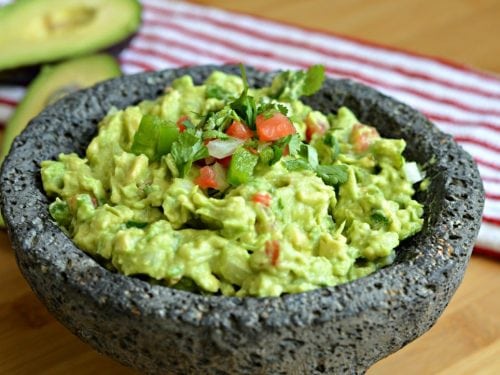This close-up photograph captures a rustic stone mortar and pestle filled with freshly made guacamole. The mortar is a dark gray, speckled, and pockmarked bowl, adding a natural and rough texture to the image. The guacamole inside is a light green-yellow hue, richly mixed with visible chunks of diced tomatoes, white onions, and jalapeno peppers, alongside generously sprinkled chopped cilantro. The scene is set on a light brown wooden table, adorned with a red and white striped towel draped diagonally in the background. A halved avocado, its pit removed, rests off to the side, subtly complementing the main focus of the rich and vibrant guacamole in the stone bowl.